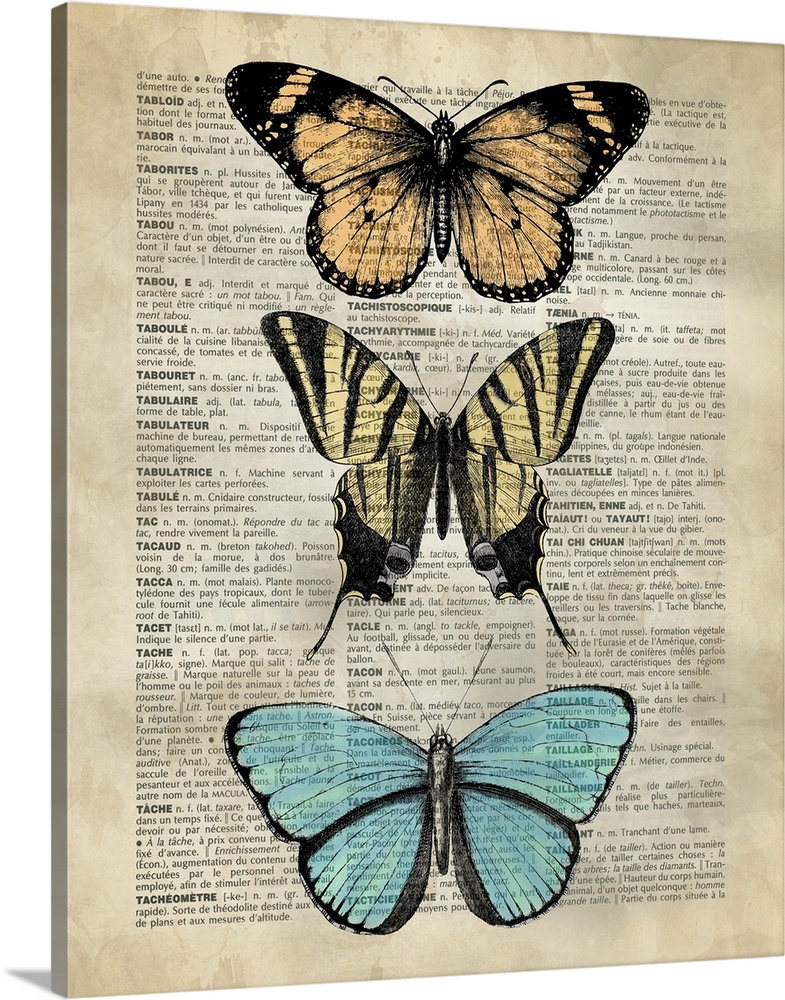This color illustration, in portrait orientation, features a detailed and striking composition of three watercolor butterflies meticulously painted on what appears to be an aged page from a dictionary. The off-white, creamy brown paper, filled with black printed text, is mounted on thick cardboard against a white backdrop. The dictionary page prominently displays entries starting with the letter "T," including words such as "tabloid," "Takara," and "taka." The butterflies are aligned vertically down the center of the page, each with distinct colors and patterns. The top butterfly is reminiscent of a monarch, showcasing vibrant orange wings with black tips. The middle butterfly is a striking yellow and black swallowtail, characterized by its zebra stripes and long, tapered lower wing points. The bottom butterfly is a serene light blue, with wider top wings and more narrow lower wings. The overall effect gives the impression of the butterflies being pressed between the pages of the book, blending natural beauty with the texture of an antique dictionary page.